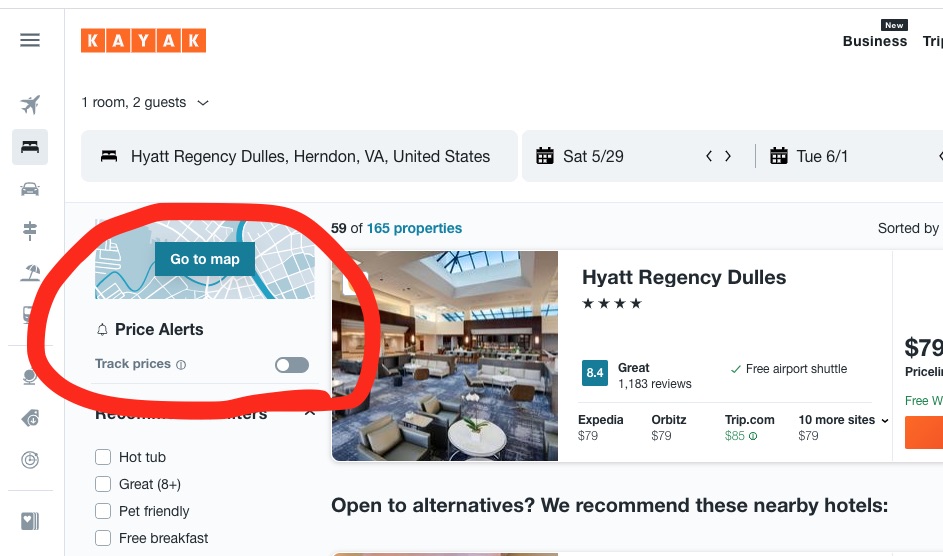In this detailed screenshot from Kayak, we see a search interface in the upper left corner displaying the travel details: "One room, two guests." Below that, there is a search bar that says "Hyatt Regency Dulles, Herndon, Virginia, United States," accompanied by a calendar icon. The dates indicated are "Saturday, 5/29" for the check-in and "Tuesday, 6/1" for the check-out.

A red circle has been added around specific options such as "Go to Map," "Price Alerts," and "Check Prices," with the latter being turned off in this screenshot. At the top of the search results, it says "59 of 165 properties" with the highlighted option being the Hyatt Regency Dulles. This property is rated four stars with an 8.4 "Great" rating based on 1,184 reviews.

The listing highlights the availability of free airport shuttles and presents various pricing options: $79 on Expedia, $79 on Orbitz, and $85 on Trip.com. There is also an indication of prices from ten more sites available through a dropdown menu. The prominently shown price beneath these details is $79.